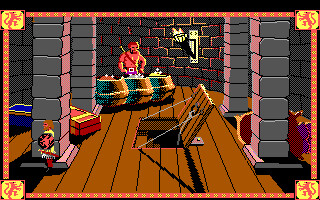The image depicts a pixelated video game scene with a meticulously detailed interface. Surrounding the central content are four orange bars, one on each side of the image — at the top, right, bottom, and left — each adorned with a distinctive yellow pattern. At each corner of the frame, there is a yellow square, all consistent in design, featuring a red and orange line that appears to form an intricate pattern.

Inside the frame, the setting appears to be a room with a wooden floor, rendered in pixel art style. A central character stands facing left, distinguished by a yellow shirt or possibly a shield emblazoned with a red line. This character also has a black and red shield, along with characteristic hardware like a sword strapped to their back via a chest strap, purple pants, and a white buckle. Positioned in front of this figure are three barrels: the one on the left contains brown powder, the one in the center is silver, and the one on the right is gold. 

In the back right section of the room, a torch is affixed to the wall, casting light across the scene. At the center of the room, an open hatch leading downstairs is visible, held open by a set of wires, contributing to the adventure or exploratory ambiance of the room. Overall, the image conveys a rich and engaging setting, evocative of classic role-playing video games.